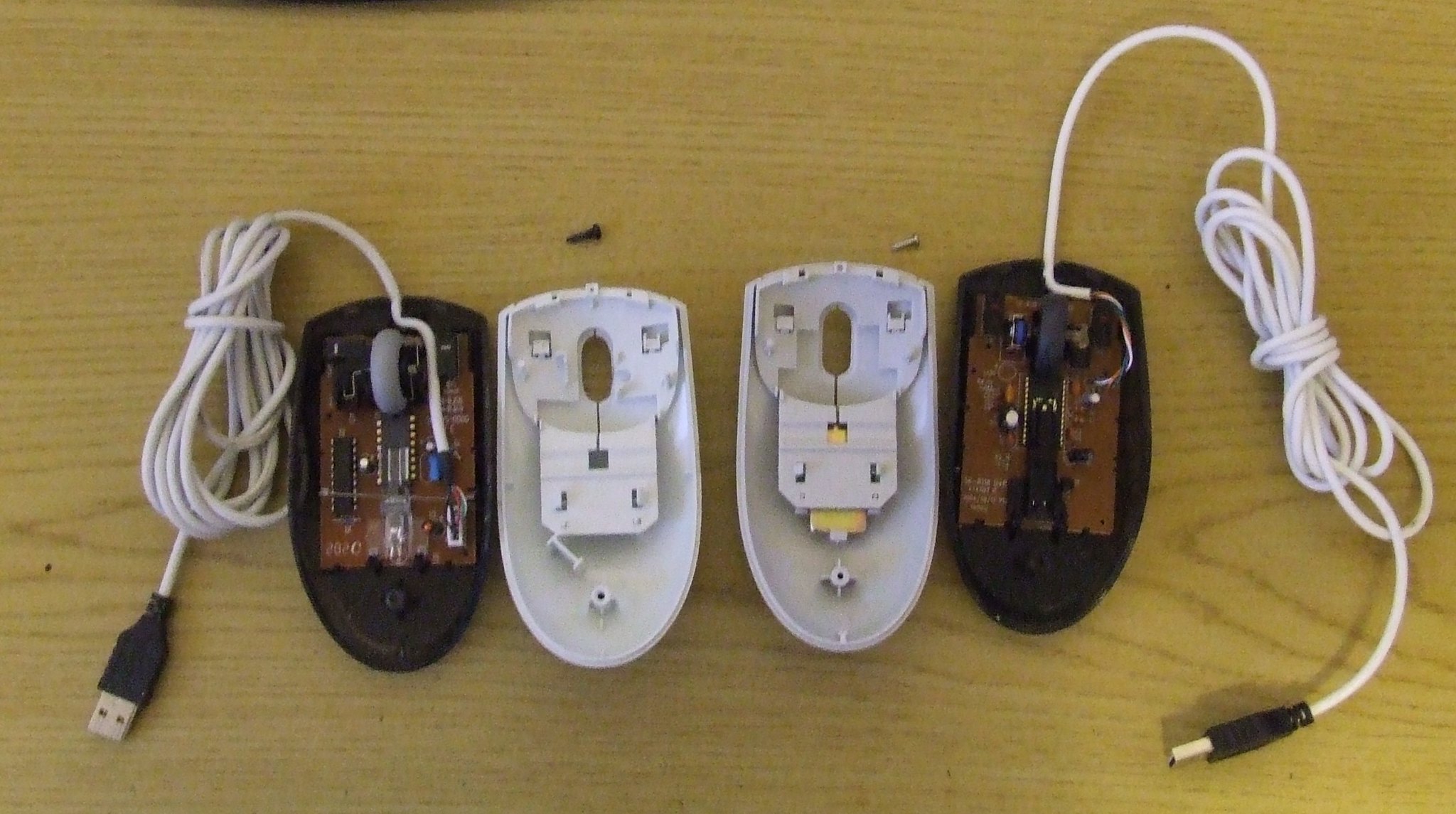This photograph captures a top-down view of a light brown wooden table with a textured pattern, illuminated softly from the bottom right corner. On the table, there are four disassembled computer mice arranged in pairs. The two outer mice have black bottoms and white tops, while the two inner mice are entirely white. Each mouse has its top casing removed and placed beside it, revealing the internal circuitry, including brown circuit boards and scroll wheels. There are neatly wrapped white USB cords extending from the black mice at the ends. Several loose screws are scattered across the tabletop. The shadow of the person taking the photo is faintly visible projected onto the table.